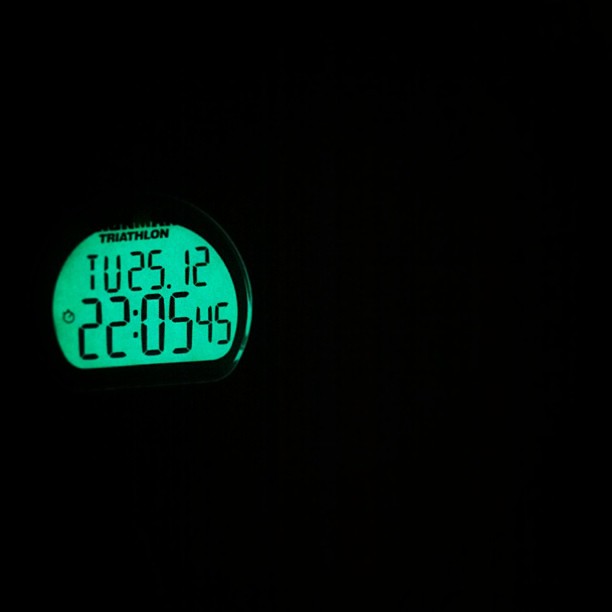In this image, a luminous green watch face or stopwatch emerges from an entirely black background, suggesting it was taken in a darkened room or an outdoor area devoid of any light. The glow of the face, reminiscent of an illuminated LCD screen, displays crisp black numbers reading "220545," which likely indicates the time. Above this numerical display, the word "Triathlon" is prominently featured, possibly denoting the brand or model of this timing device. The stark contrast between the vibrant green glow and the pitch-black surroundings creates a striking visual focus on the watch face.